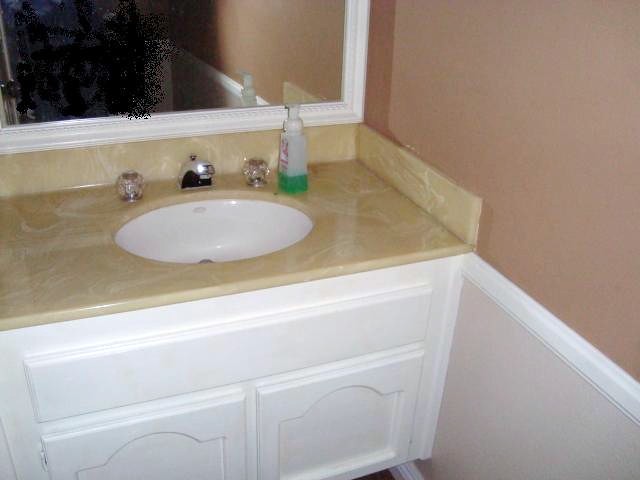The image showcases a bathroom counter with a light beige to light brown surface. The counter features silver faucets. Placed on the counter is a plastic bottle that is less than half full with green liquid soap, topped with a white pump for dispensing the soap. 

Above the counter is a white-framed mirror. Inside the mirror, a black shadow is visible in the background. Below the counter, there is a white cabinet area, consisting of two white cabinet doors. Each door has an arch-shaped design at the center. Subtle off-yellow accents are scattered throughout the white cabinetry.

To the right of this setup, the lower portion of the wall is painted light pink, transitioning to a muted brick red color at the top. A white decorative horizontal rectangle separates these two colors, running down the right side of the wall. The mirror reflects a black shadow to the left side, with no other discernible details.